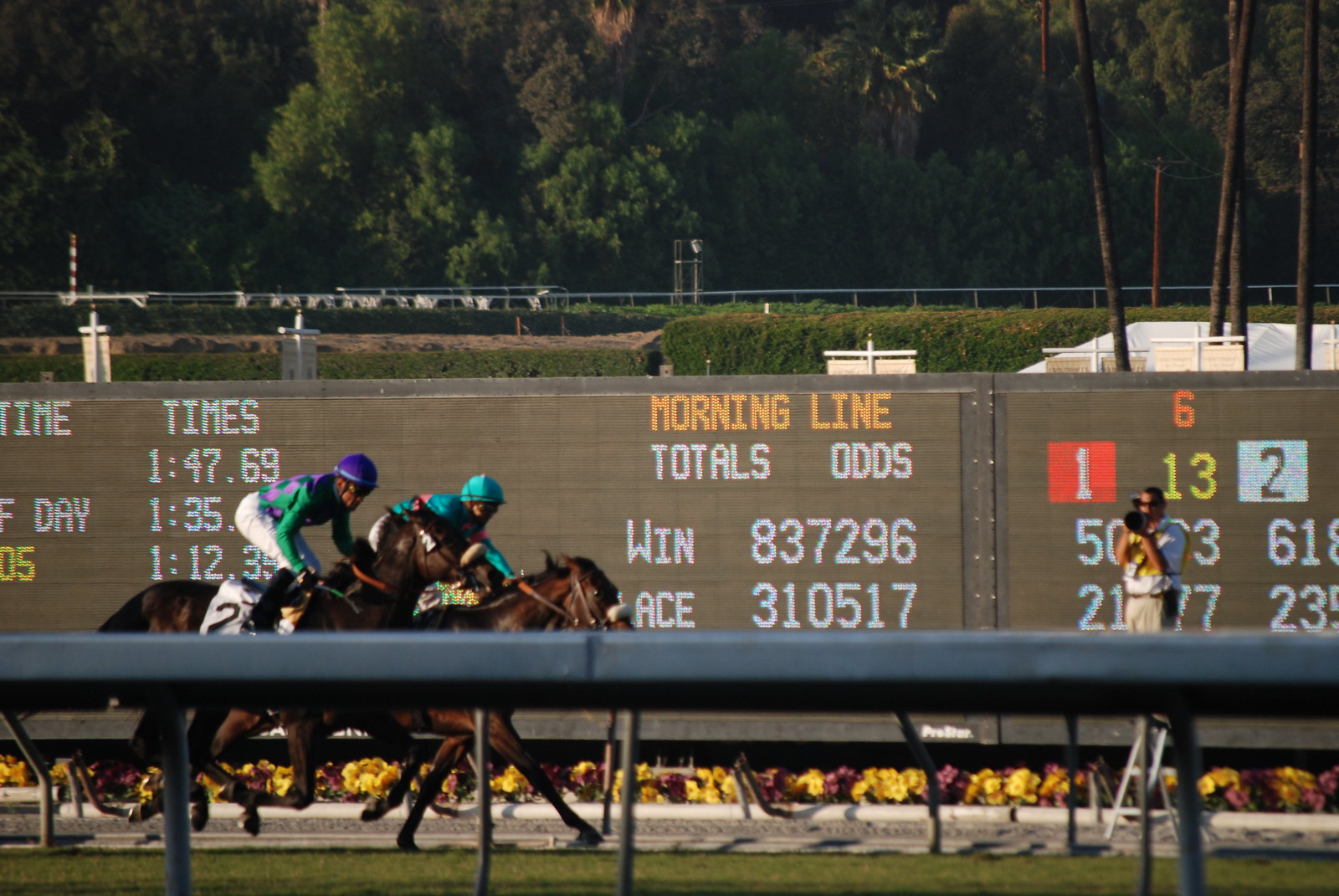The image captures a thrilling moment in a horse race, viewed from a ground-level vantage point just outside the fence, which runs along the bottom half of the scene. Two jockeys, mounted on brown horses, are racing neck and neck, speeding past an electronic scoreboard that displays various race details like odds and times. The jockey in the lead sports a teal jersey and matching cap, while the one trailing wears a blue and green outfit. They're about to cross the finish line, as evidenced by a photographer in the background, positioned on a stepladder and ready to capture a photo finish. The photographer, clad in a white shirt and khaki pants, holds a black camera. Behind the track, a lush backdrop of trees and shrubs suggests a pleasant summer day. The digital scoreboard prominently shows figures such as odds and winnings, with detailed categories like "Win" and "Ace," alongside an array of figures denoting times and other statistics. This dynamic moment epitomizes the excitement and precision of competitive horse racing.